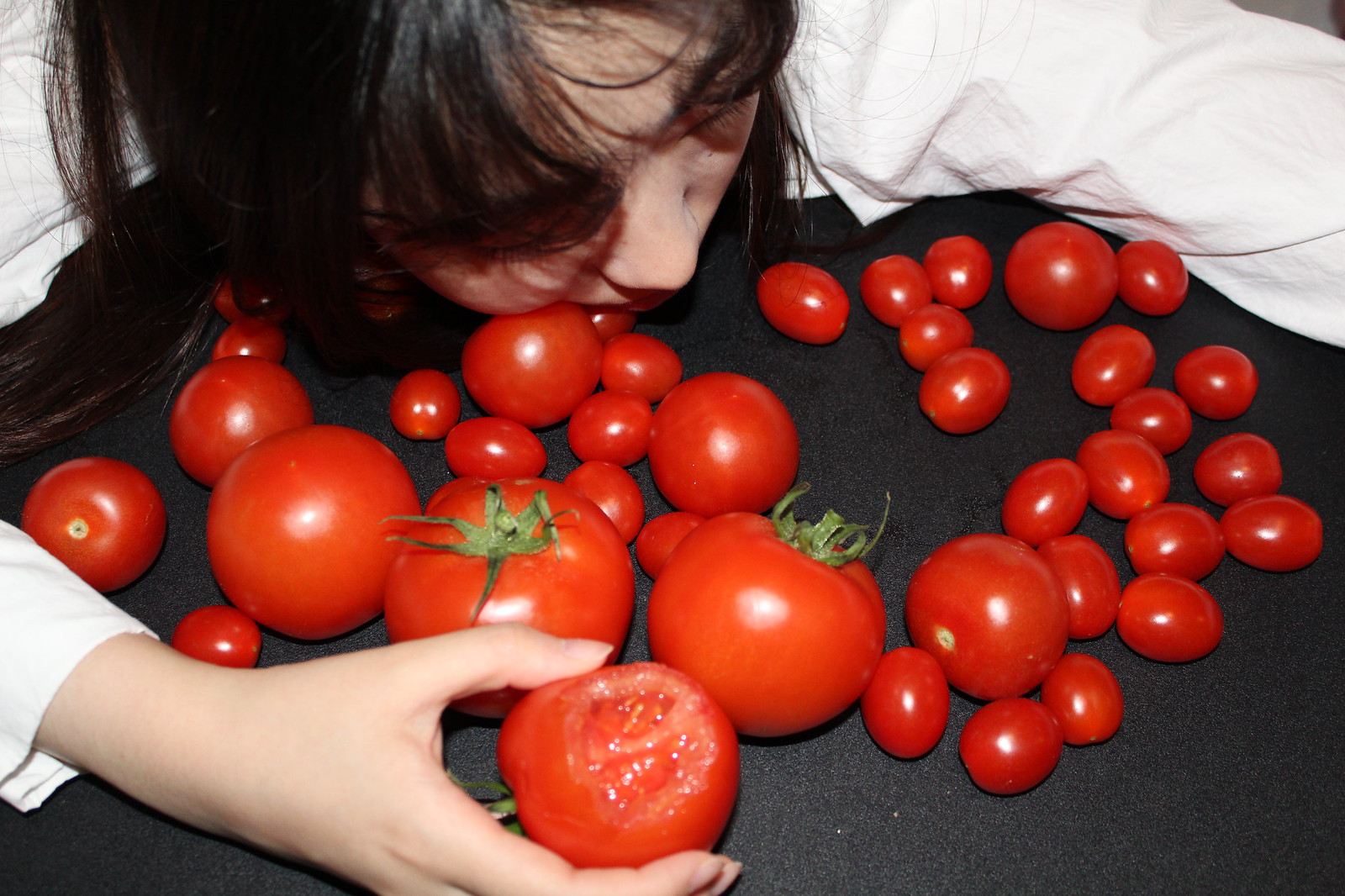In the image, there is a close-up of a woman with black hair and black fringe bangs, wearing a white long-sleeve shirt. She is leaning over a black surface, possibly a table, filled with a vibrant assortment of tomatoes. These include small cherry tomatoes, slightly larger grape tomatoes, and three full-sized tomatoes, two of which still have their green leafy tops. The woman is embracing the tomatoes with both arms, almost as if she is hugging them, with her face gently resting on top of a few. In her right hand, she holds a tomato with a bite taken out of it, showcasing its juicy interior. The scene is a tender and intimate portrayal of her affection for the fresh produce.